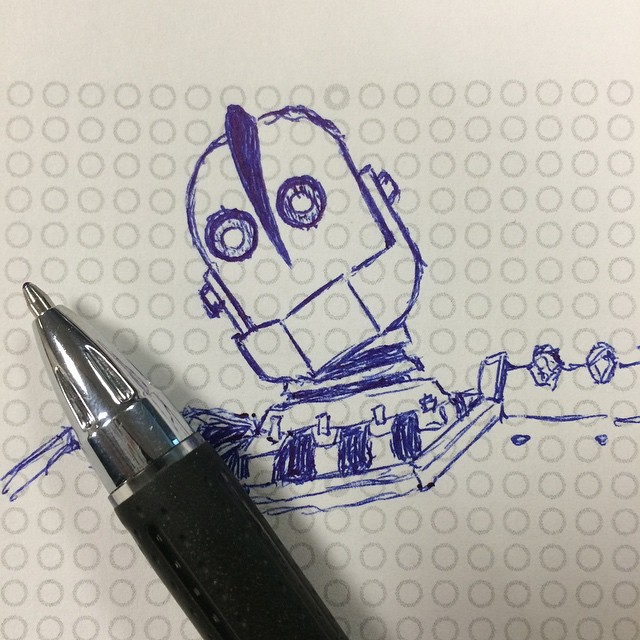This image features a meticulously detailed pen drawing on a small piece of white paper, entirely covered in closely spaced, perfectly aligned gray circles, except for a half-inch margin at the top. In the center of the paper, a robot is depicted with its head tilted to the left. The robot's head has rivets on either side, and a prominent blue fin runs from the top of its head down to its nose. The robot's eyes are round with white pupils, giving it a lifelike appearance. Its mouth, featuring a cut that suggests an articulating jaw, is currently closed but hints at possible movement. The robot's neck is adorned with dark blue banding, seamlessly transitioning into the top of its shoulders, which also feature additional rivets. A black pen with a silver cap is intrusively present in the middle foreground, extending upwards to the left midsection of the image, hinting at the tools used to create this blue ink drawing.